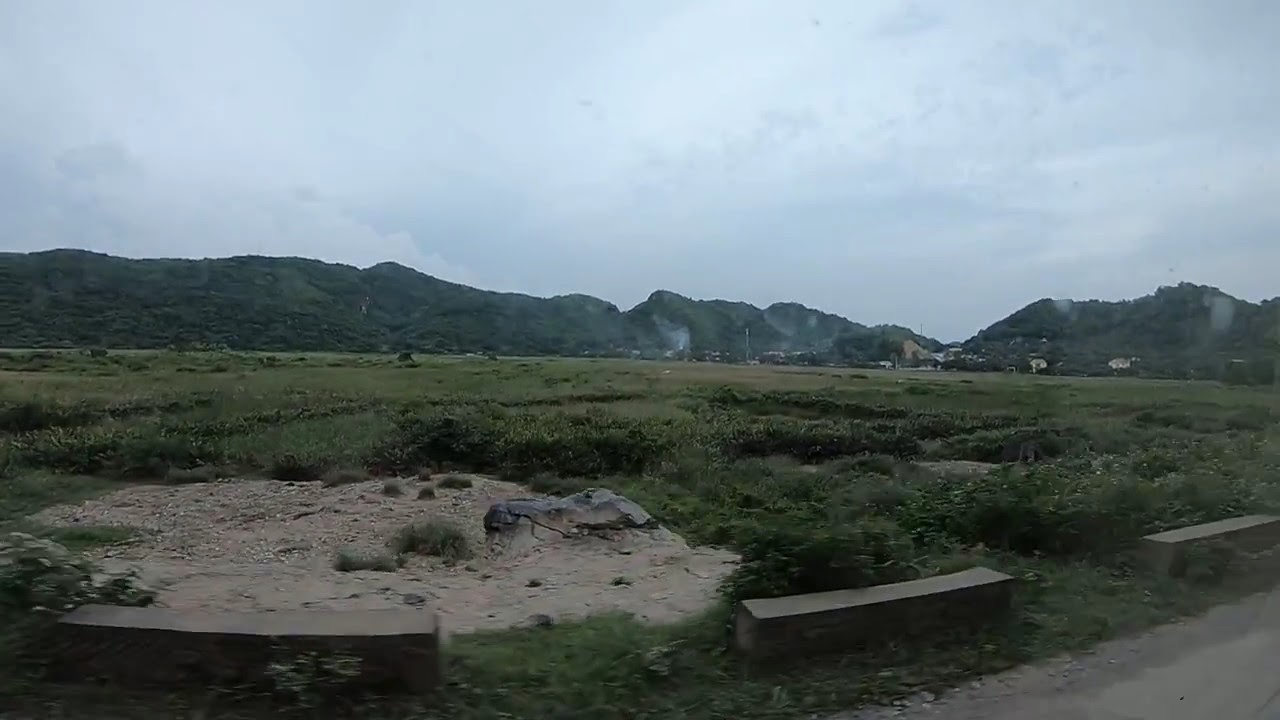The photo captures a roadside scene under an overcast sky, suggesting a dreary or possibly rainy day with no visible sunlight. The lower right corner features a tan dirt road bordered by rectangular cement pillars, which mark the road's side and end. In the foreground, there is a bare patch of brown dirt on the left side and a large green field filled with vegetation in front of us. This field extends into the background where small hills, also covered in green vegetation, rise up. At the base of these hills, rectangular buildings can be seen. The sky is filled with dark and light gray clouds, enhancing the gloomy atmosphere. Various antennas are visible within the town situated at the foot of the hills.